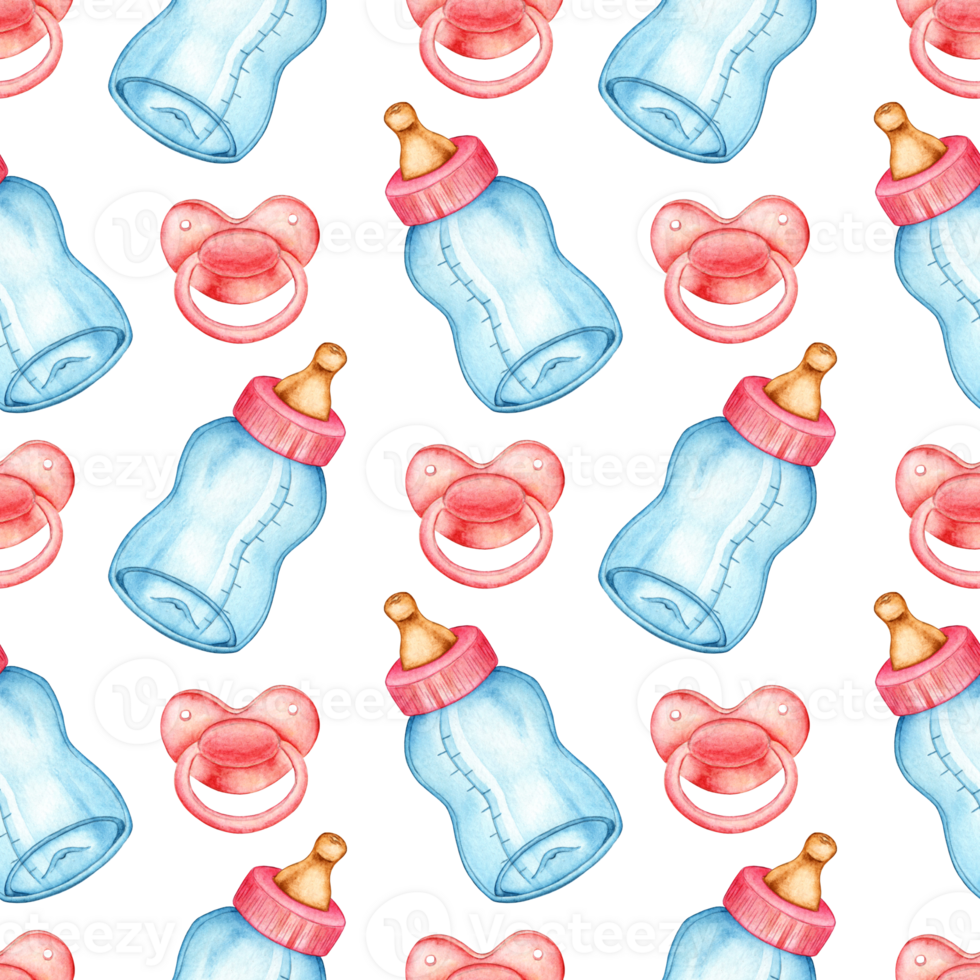This image, styled as a digital drawing on a white background, features a repeating pattern commonly used for digital paper or tiles. It depicts blue baby bottles with pink lids and brown nipples, interspersed with pink heart-shaped pacifiers with circular pull rings and ventilation holes. The baby bottles, detailed with faint measurement lines, alternate diagonally at 45-degree angles—some slanting to the upper right and others to the upper left. The pacifiers and bottles are arranged in parallel lines, creating a consistent and alternating pattern throughout the graphic. Some elements are cut off at the edges, indicative of a tiled design meant for larger applications. Subtle, almost hidden text "VECTEEZY" overlays the image in light gray, accompanied by a small circular logo with a 'V'.